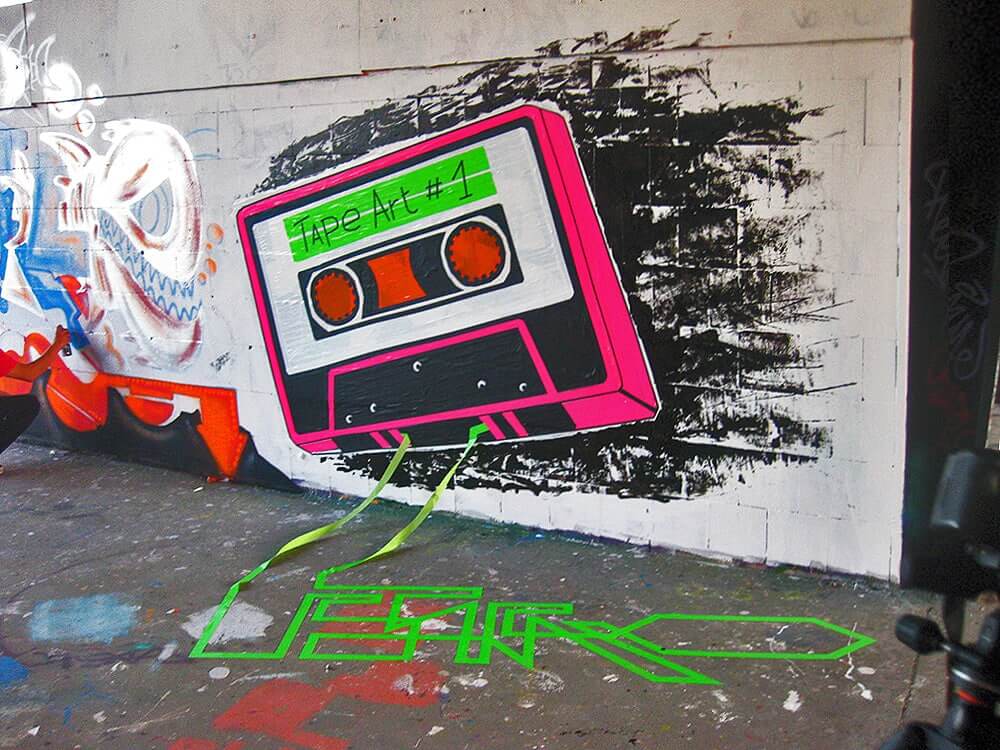The scene captures a vibrant mural on a white cinder block wall, illustrating a large, neon pink and black cassette tape with a strikingly 80s vibe. The tape, labeled "Tape Art Number One" in black letters on a highlighted green box at the top, is the mural's centerpiece. Descending from the tape, a vivid green string extends in a realistic, 3D manner, trailing onto the ground and forming an intricate yet illegible word on the concrete. The mural's background is predominantly black, enhancing the tape's vivid colors. To the left side of the tape, additional graffiti features white text and an abstract shape resembling a shark with sharp teeth and fin-like protrusions, adding another layer of artistry to the scene.